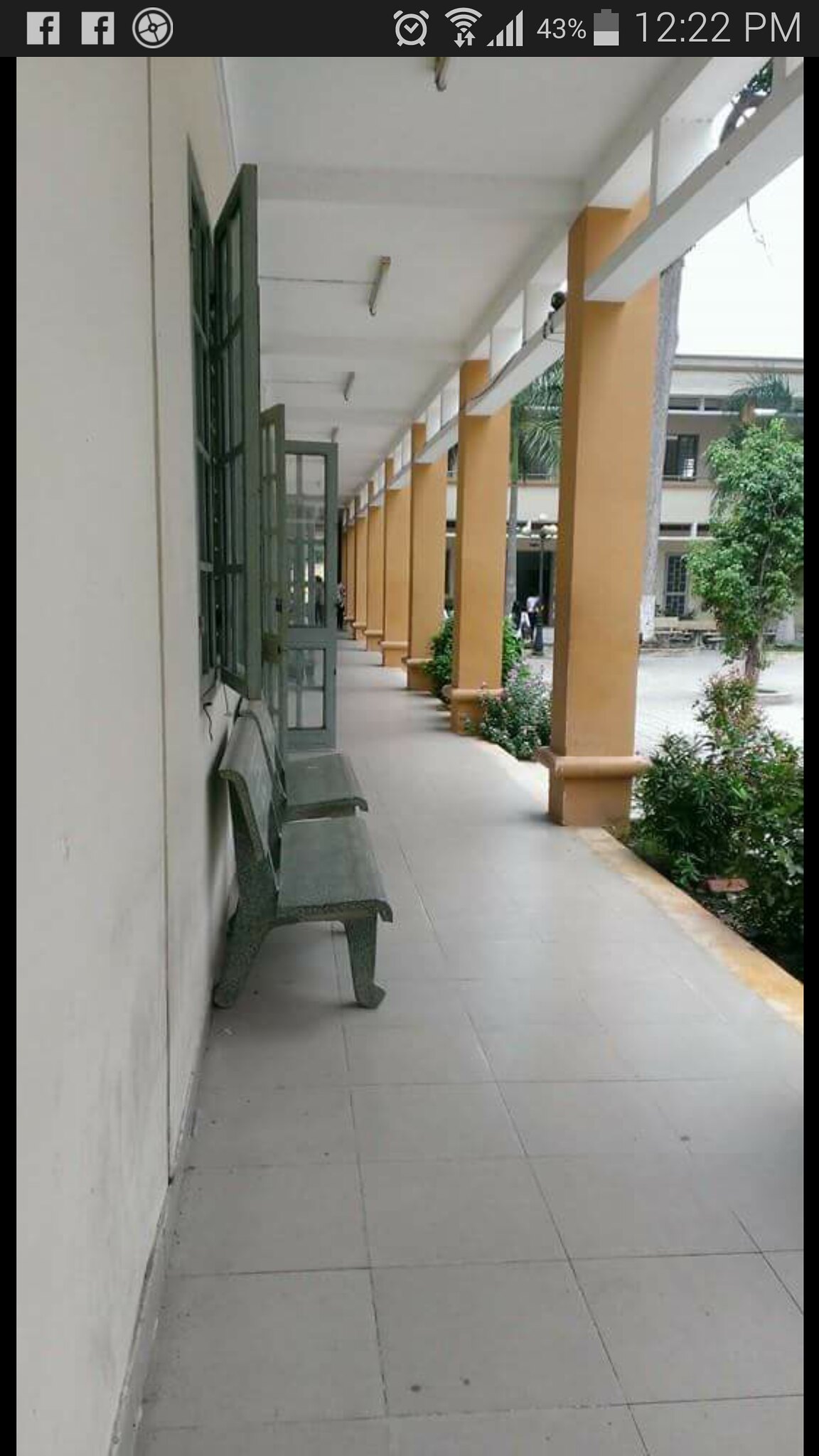The image captures the exterior of a well-maintained building, reminiscent of a Californian school or perhaps a resort. The screenshot is taken from an Android phone, indicated by various icons: two Facebook logos, a steering wheel icon, an alarm, Wi-Fi, cellular signal indicators, and a 43% battery at 12:22 PM. The building features several design elements: predominantly white walls with lighter green accents on the window frames, doors, and benches. The ground is lined with gray concrete tiles interspersed with green shrubs and trees, giving the area a refreshing look. Yellow pillars stand out against the building, and brown columns with white bars extend from the ceiling. There are also tan columns with white beams supporting a white overhang, underneath which fluorescent lights are visible. The background reveals more of the same building, maintaining a cohesive aesthetic with the foreground.